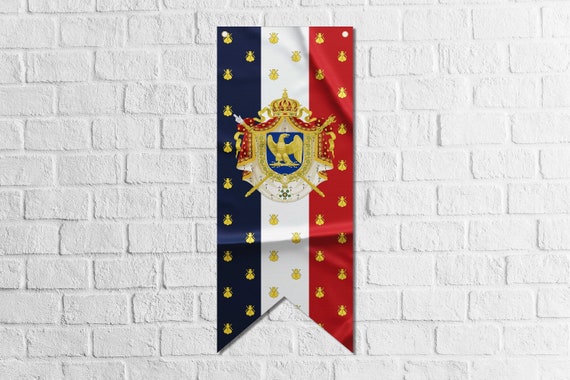This is a photograph of a vertical rectangular banner hanging on a white painted brick wall. The banner features a trio of stripes in blue, white, and red, adorned with numerous small gold designs repeated throughout. Its bottom edge is notched, resembling a split pennant with two tongues. Centrally positioned within the banner is an ornate coat of arms that exudes a European flair, predominantly in gold and red hues. The coat of arms includes a gold shield with an eagle bearing a branch in its talons, crossed by a scepter and a sword. The shield is topped by a crown, from which a red banner or curtain seems to drape down the sides. Additional golden emblems, which might resemble bees, are evenly distributed across the stripes in nine rows, creating a detailed and intricate pattern. The bottom of the banner is also accented with white filigree decorations.